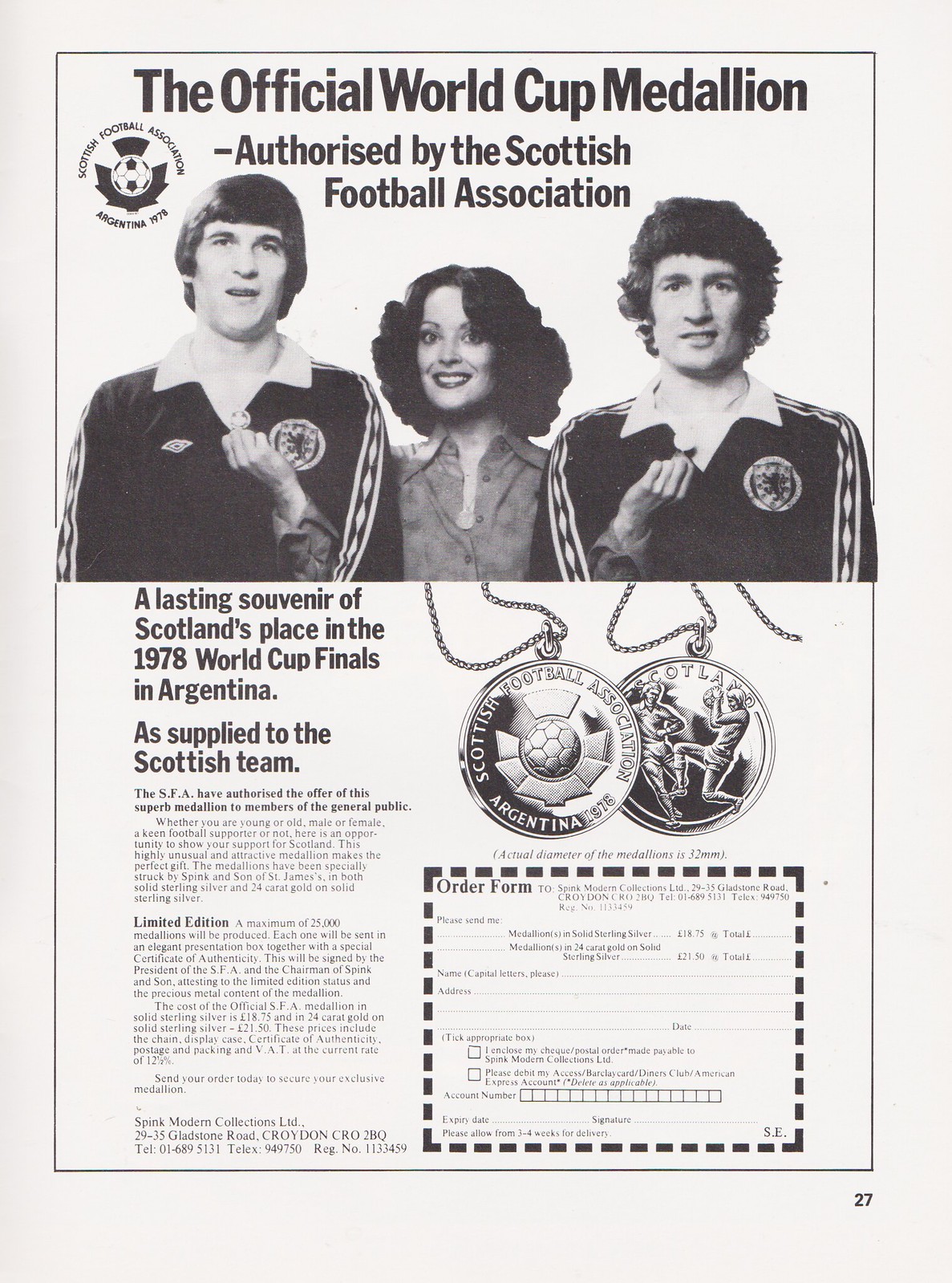This image appears to be a page from a magazine or program, specifically advertising a limited edition medallion authorized by the Scottish Football Association commemorating Scotland's participation in the 1978 World Cup Finals in Argentina. At the top, there is a black and white photograph showing three people standing side by side: a man on the left and another on the right, both dressed in tracksuits, with a smiling woman in the middle who has her hands up to the collars of the men’s shirts. Above this image, bold text declares "The Official World Cup Medallion Authorized by the Scottish Football Association." Below the photograph, there is a detailed advertisement. On the left side, against a white background, it reads: "A lasting souvenir of Scotland's place in the 1978 World Cup Finals in Argentina as supplied to the Scottish team." Further down, there are paragraphs elaborating on the medallion's offer. On the right side of the page, there are two black and white images of the medallions, each on chains. The medallion features two distinct sides: one side has the text "Scottish Football Association, Argentina 1978" encircling a soccer ball, while the other side depicts two soccer players with the word "Scotland." At the bottom of the page, there is an order form for those who wish to purchase the medallion, to be mailed to Sphinx Modern Collection Ltd, 2935 Gladstone Road, Croydon CRO2 BQ, including a telephone and telex number for contact.